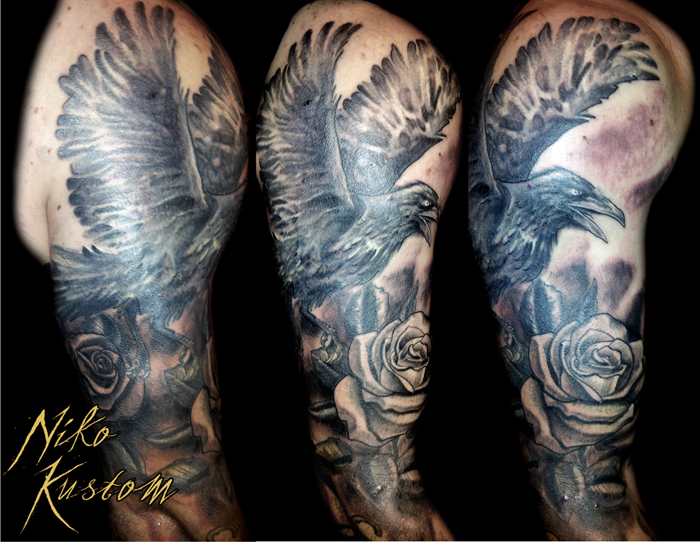The advertisement image showcases a black and white tattoo on a single person's right arm, presented from three different angles—back, side, and front—primarily depicting the shoulder to the elbow. The person, wearing a black tank top, has fair skin, and the tattoo features a black bird, likely a crow or raven, with upswept wings and an open beak revealing an angry eye. This bird is perched above a large, intricate rose, detailed with contrasting shades of black and gray, extending down to a stem with leaves. The text "Niko Custom," spelled N-I-K-O-K-U-S-T-O-M, is prominently displayed in yellow letters in the bottom left corner against the predominantly dark background.